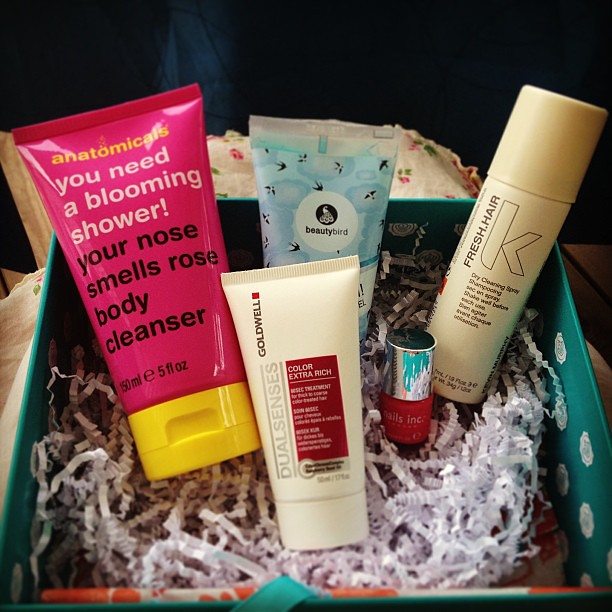In the dimly lit ambiance against a dark background, an elegant green gift box adorned with delicate white designs sits proudly on a table. Possibly behind the table, an indistinct chair adds a subtle depth to the scene. The box is a treasure trove of luxurious body grooming products, showcasing five distinct items. 

The centerpiece is a generously sized body cleanser labeled "Your Nose Smells Rose," encased in a vibrant magenta packaging. Towering next to it is a sleek blue tube embossed with "Beauty Bird." In the foreground, a bright yellow tube with a dark reddish square commands attention, hinting at an "Extra High" product. Adding a touch of classic elegance, a vivid red lipstick lies beside them. Completing this exquisite collection is a fresh hair freshener encapsulated in a stylish aerosol can. Each product stands poised, inviting indulgence and self-care.